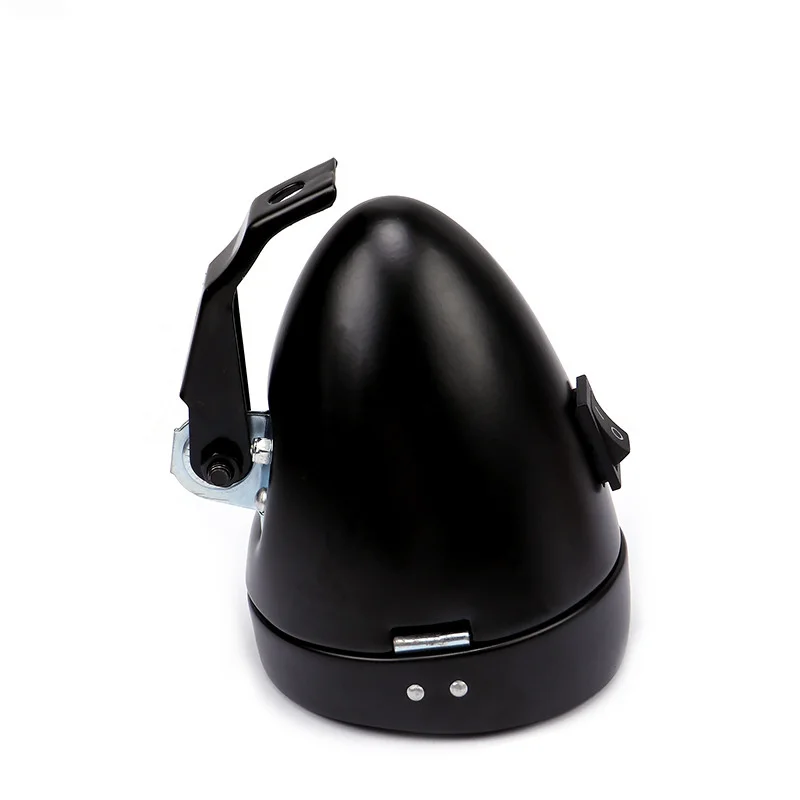The image features a sleek, black, egg-shaped object with a flat base, centered against a white background. The top portion resembles a long, thin dome, with a flat base. On the right-hand side, midway up, there is a power button resembling a switch marked with a white line and a white circle. The base includes a stainless-steel folding flap with two small metal circles and a hinge mechanism, allowing the top to separate from the base while remaining attached. On the left-hand side, a stainless-steel attachment connects to a black arm that protrudes straight up and angles to the right, stopping above the top of the egg. This black arm has a hole through it. The contemporary design integrates black and stainless-steel elements, giving it a modern and functional appearance, potentially indicative of a device that can open and close, with the arm possibly serving as a handle or a stand.